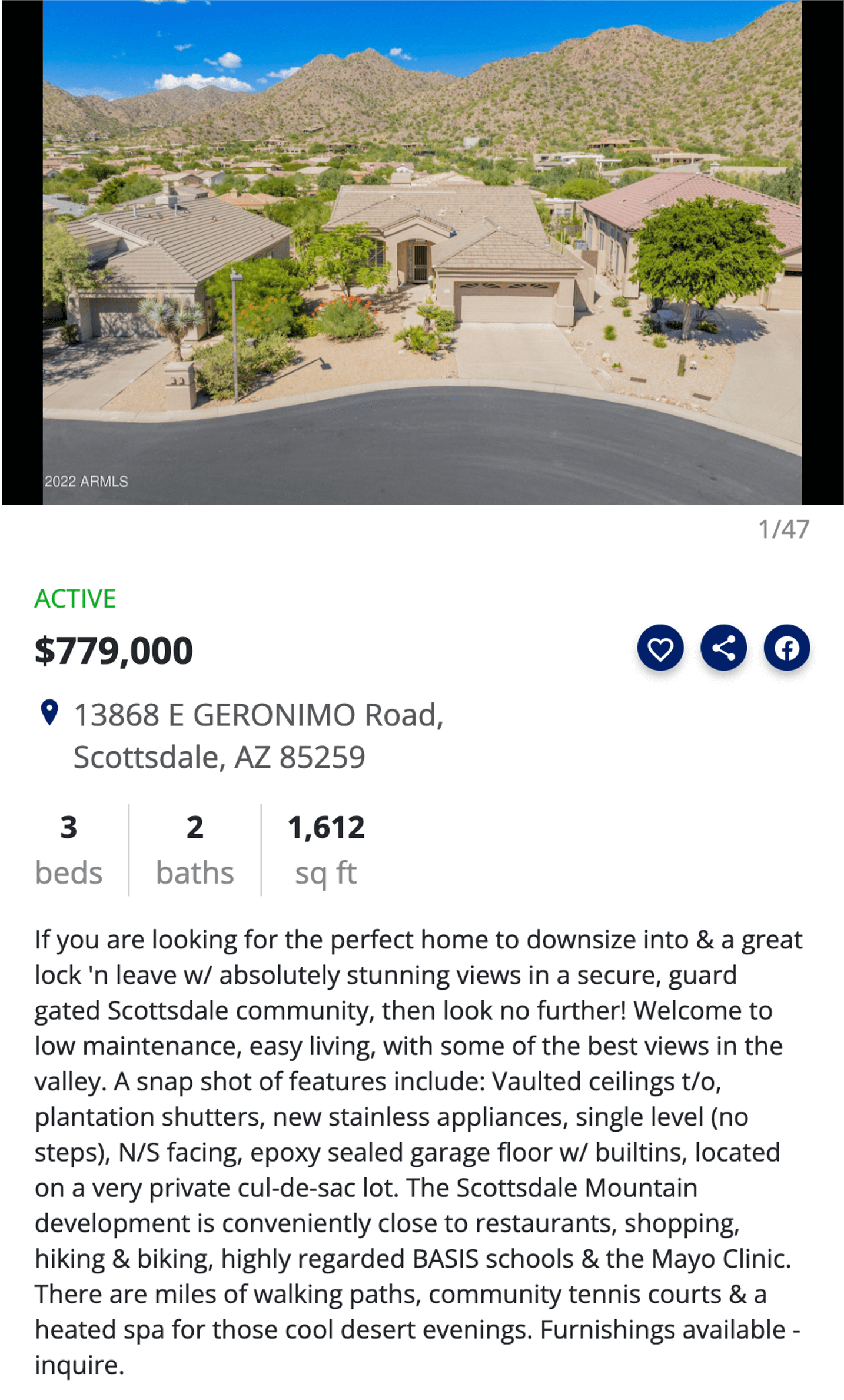**Detailed Caption:**

This screenshot is taken from a real estate website similar to Zillow or Trulia. At the top, there's a slightly aerial daytime photograph showcasing the property listed for sale. The image captures a single-story house situated in a desert area, highlighting its tan exterior and roof, which seems to be either painted or made from tan stone or siding. The house features one garage conveniently close to the road. The picturesque background consists of rocky, tree-covered mountains under a partly cloudy blue sky. In the foreground, the house is part of a quiet neighborhood with two other single-story houses on either side.

Below this captivating image, a green capital-lettered "ACTIVE" status indicates that the property is currently on the market.

The asking price of the house is prominently displayed in bold black text at $779,000, accompanied by three icons for liking, sharing, and Facebook.

Further details include the address, 13868 E Geronimo Road, Scottsdale, Arizona 85259. The property specifics follow, listing three bedrooms, two bathrooms, and a total living space of 1,612 square feet in black and gray lettering.

A detailed paragraph describes the property, emphasizing its suitability for downsizing and offering "lock and leave" convenience within a secure, guard-gated Scottsdale community. The home promises low-maintenance, easy living with stunning valley views. Key features mentioned are vaulted ceilings, plantation shutters, newer stainless steel appliances, single-level layout devoid of steps, north-south orientation, and an epoxy-sealed garage floor with built-ins. The property is situated on a private cul-de-sac lot within the Scottsdale Mountain Development. This prime location is close to restaurants, shopping, hiking, and biking trails, highly regarded BASIS schools, and the Mayo Clinic. Residents can enjoy miles of walking paths, community tennis courts, and a heated spa for those cool desert evenings. Furnishings are available upon inquiry.